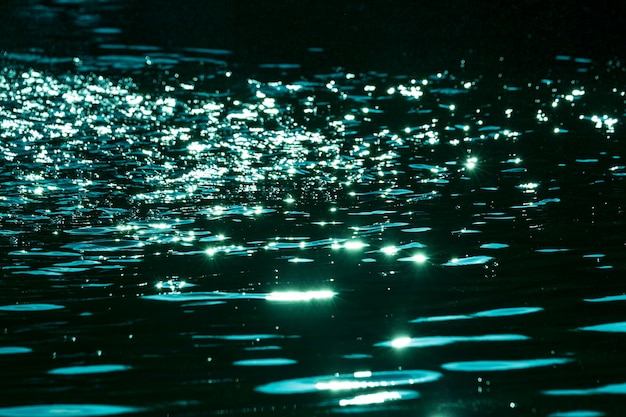The photograph captures a scene of water under a light source that creates a shimmering, dotted effect across its surface. The quality of the image is notably poor, making it difficult to discern exact details about the environment or time of day. The water appears in varying hues, described differently by various observers—ranging from a dark, almost blackish blue to a slimy green or even a neon teal. The scattered light reflections, which could be from the sun, moon, or artificial sources, add to the mysterious and almost surreal atmosphere with their beaming white, light yellow, and neon green tints. The water is still, with no waves, figures, or objects visible, presenting a solitary and enigmatic scene. The photograph is 3 by 5 inches with no date, text, or distinguishing features beyond the reflective and glistening water surface.